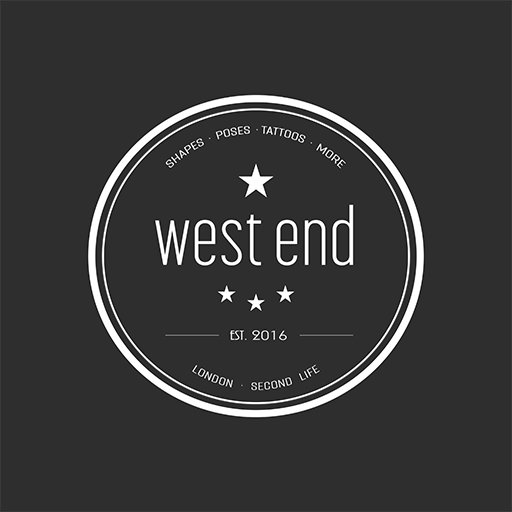The image is a square graphic design with a black (or dark gray) background featuring a circular white border enclosing all elements. At the top of the circle, it reads "Shapes, Poses, Tattoos, More" in white letters, followed by a single white star beneath. Centrally within the circle, the brand name "West End" is prominently displayed in white font. Below "West End" are three small white stars, and further down, it reads "Established 2016." At the bottom within the circle, the text "London Second Life" is also in white. All text and graphics are in white against the dark background, giving the entire design a high-contrast appearance. The overall feel suggests that it could be a logo, poster, or advertisement for a business related to shapes, poses, tattoos, and more, established in 2016 in London.